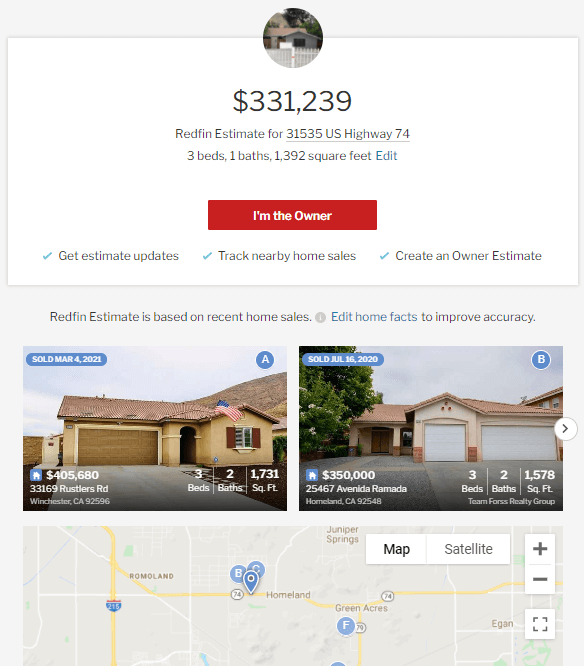An image detailing various real estate information and estimates from Redfin:

At the top, a prominent Redfin estimate of $331,239 is displayed for a specific address. This estimate pertains to a single-family home featuring three bedrooms, one bathroom, and a total area of 1,392 square feet. Below the estimate, there is a red rectangular background with bold white text stating, "I'm the owner."

Further below, there are three selectable options, each marked with a blue checkmark to the left. They read: "Get estimate updates," "Track nearby home sales," and "Create an owner estimate." Additionally, text indicates that the Redfin estimate is based on recent home sales, and users can edit home facts to improve accuracy.

At the bottom left section, there's an image of a house that is tan-colored with a brown rooftop, listed for $405,680. This property includes three bedrooms, two bathrooms, and measures 1,731 square feet. The address is mentioned directly below the listing.

To the right, another house is depicted, featuring a tan exterior with two white garage doors and a matching tan rooftop. A tree occupies the top left corner of this section, and the sky is a gloomy gray. This property is listed at $350,000 and offers three bedrooms, two bathrooms, and covers an area of 1,578 square feet. The address along with the town and zip code are also provided.

At the bottom, there is a gray-toned map showing the location of the two houses mentioned.